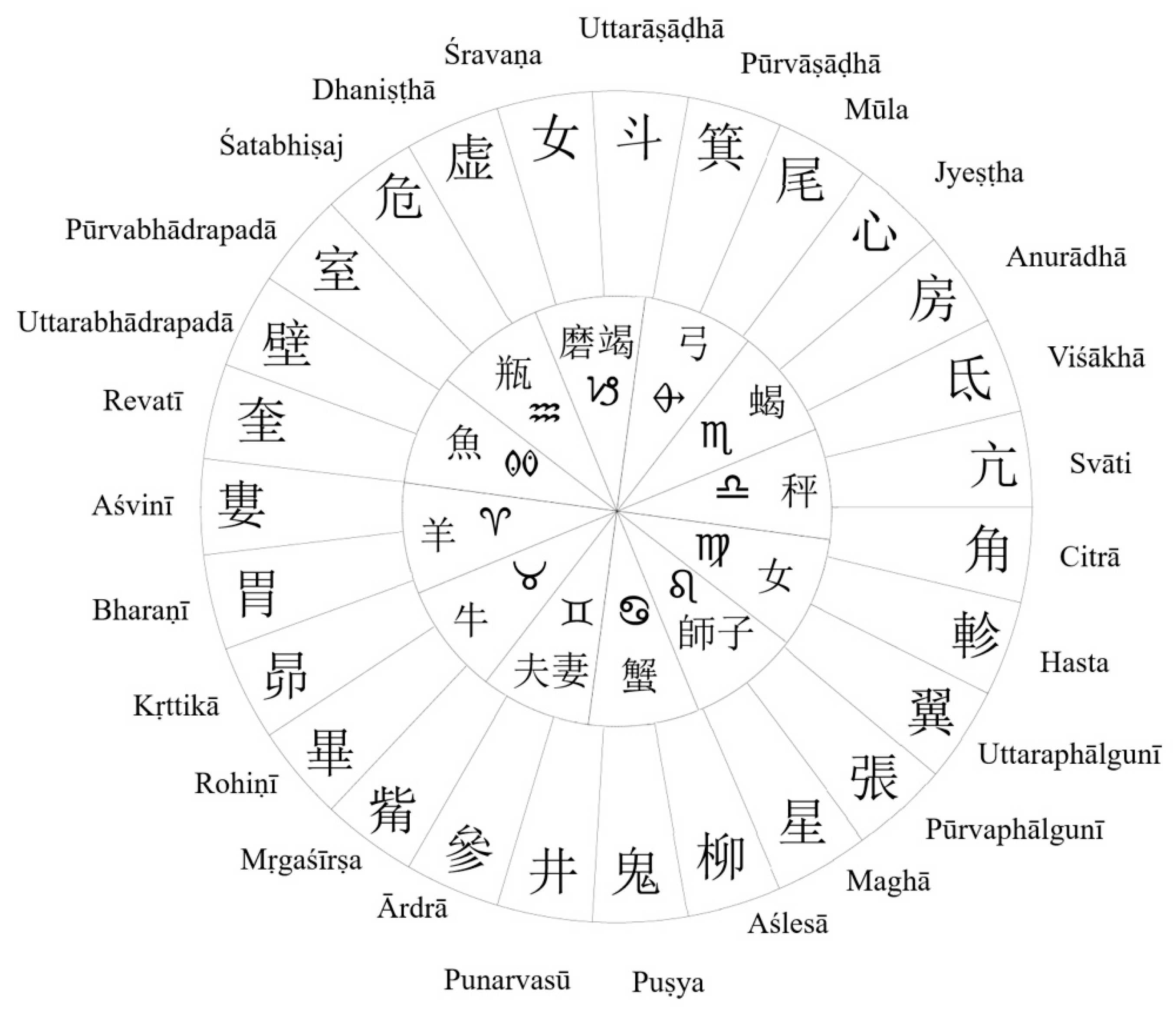This black and white circular image features intricate details within two concentric circles. The inner circle is divided into 12 triangular sections, each containing two or three symbols and smaller triangular subsections. From the center, lines radiate outwards like spokes, dividing the segments precisely. Surrounding the inner circle is a larger outer circle, also segmented, but with one symbol per section. Encircling the entire image, outside the large circle, are roughly 20 to 30 words written in a foreign language using the regular alphabet. Some of the words include "Ravati," "Asvini," "Barani," "Kritika," and "Rohini." These words and symbols suggest a format similar to that of an ancient chart or a Rosetta Stone, evoking a sense of detailed linguistic and symbolic structure.